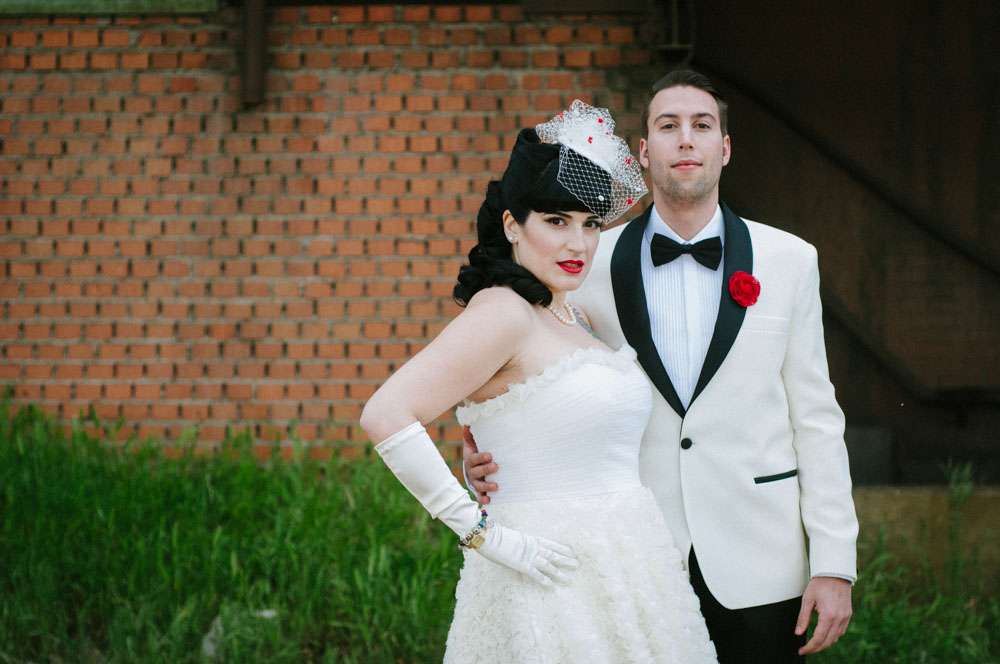The photograph captures a couple, resembling a bride and groom in a vintage-style scene, with their attire and setting evoking the early 1960s. Positioned slightly right of center, the woman, on the left, faces outward while glancing back to her right. She has black, curly hair cascading over her right shoulder, wears striking red lipstick, and adorns a black hat with a white mesh veil dotted with red pins. Her white dress flares slightly below the waist and is complemented by a white glove on her right arm, alongside a likely pearl bracelet or wrist accessory.

To her right stands the man, dressed in a white tuxedo with black accents, including a black bow tie and black pants. His white jacket features a gray lapel and is accessorized with a vivid red rose pinned on his chest. He has short brown hair and a subtle five o’clock shadow. His right arm is wrapped around the woman’s waist, and his left hand hangs by his side.

The backdrop consists of a red brick building and a lush grassy area. A stairwell with a railing is noticeably visible behind them, with steps beginning next to the man's right elbow, descending into a small cement area before the scene transitions into more greenery.